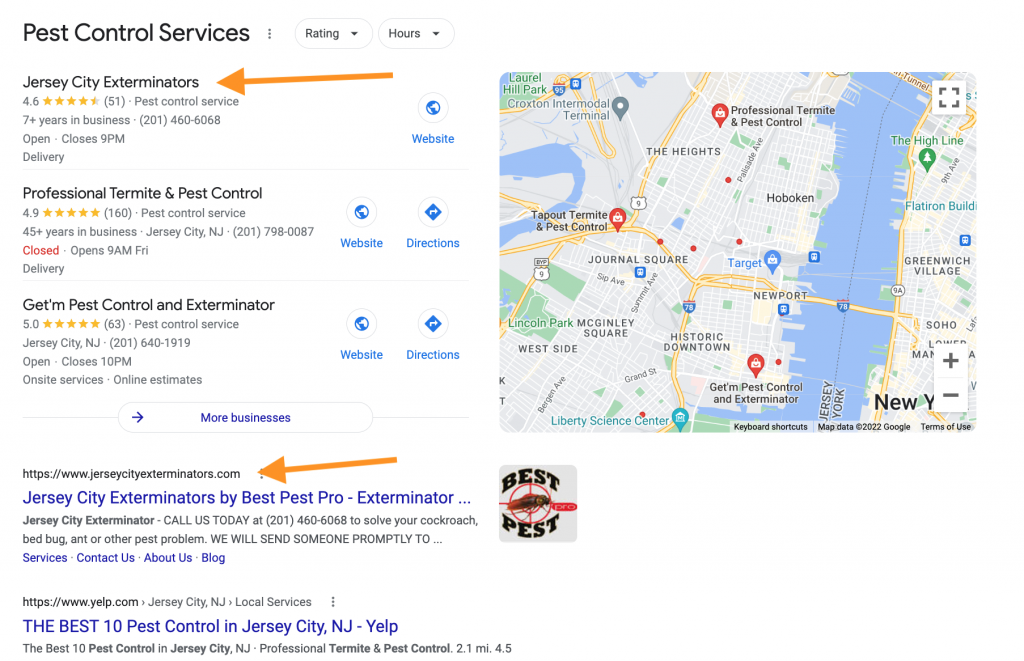In this image, a Google search result for pest control services is displayed. Although the search bar itself isn't visible, the listings of various pest control companies occupy the screen.

The first result features "Jersey City Exterminators," highlighted by an orange arrow. This service boasts a rating of 4.6 stars out of 5, based on 51 reviews. It is identified as a pest control service that has been operational for over seven years. The contact number provided is 201-460-6068. The business is currently open and will close at 9 p.m. Additionally, they offer delivery services. Users have the option to visit their website; however, directions to their physical location are not available.

The second listing is for "Professional Termite and Pest Control," which has an impressive rating of 4.9 stars out of 5 from 160 reviews. This business has been serving the community for more than 45 years. Located in Jersey City, New Jersey, they can be reached at 201-798-0087. The service is currently closed but will reopen at 9 a.m. on Friday. They also provide delivery services. For this listing, you can either access their website or obtain directions.

The third result is "Get'em Pest Control and Exterminator," with a perfect rating of 5 stars out of 5 from 63 reviews. Also situated in Jersey City, New Jersey, this service can be contacted at 201-640-1919. The business is open and will close at 10 p.m. They offer on-site services and provide online estimates. Users can opt to visit their website or get directions to their location.